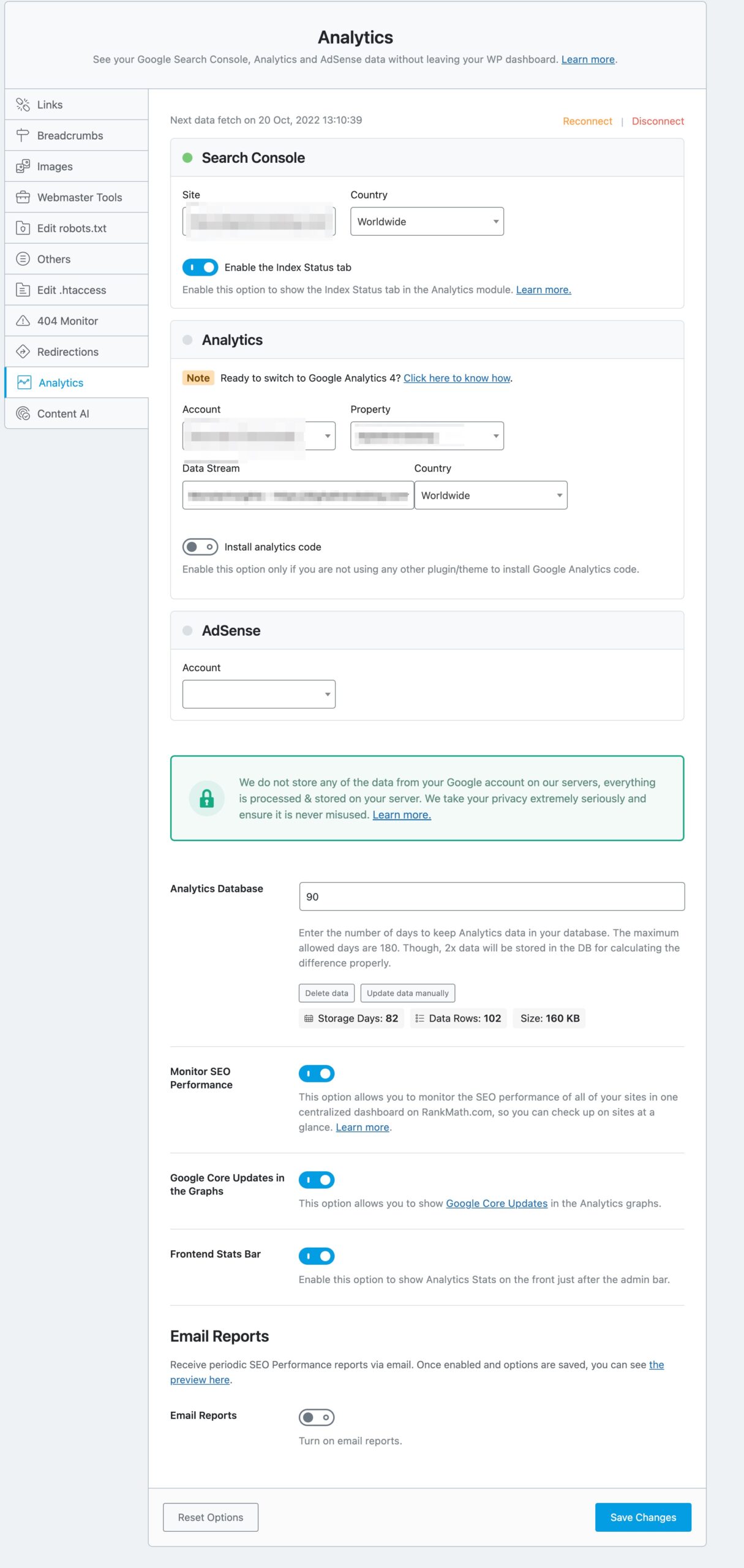**Caption:**

The image features a detailed dashboard interface for managing Google Analytics, Search Control, and AdSense data within a WordPress platform.

At the top of the image, a black text header reads: "Analytics: See your Google Search Control, Analytics, and AdSense data without leaving your WP dashboard." The word "more" is prominently highlighted in blue.

On the left side of the screen, a vertical sidebar menu lists several navigational links in black text. These links, from top to bottom, include: Breadcrumbs, Breadcrumbs Images, Webmaster Tools, Edit Report txt, Adas, Edit htaccess, 404 Monitor, Redirection, Analytics, and Content AI. Notably, the 'Analytics' link is highlighted.

To the right of the sidebar, the interface displays the analytical data section. It shows:

- "Next data fetch on 20 October" with options to reconnect or disconnect.
- A section labeled "Search Control" indicating the site is targeting the "Worldwide" audience, marked with an enabled blue icon.
- A sub-section of "Analytics" showing details like account property, data stream, country (worldwide), and an option to "Install an analytics code." This option is currently toggled off with a suggestion to enable it if no other plugin is used.

Below this, an "AdSense" account section states that the account is not inserted. A green text message reassures users about data privacy, stating: "We do not store any data from your Google account on our servers. Everything is processed and stored on your server. We take privacy extremely seriously and ensure it's never misused." The text is bordered in green.

Further down, the analytic database is shown to be 90% complete. Other toggle switches displayed include:
- "Monitor SEO performance" (ON)
- "Enable click or update graphs" (ON)
- "Frontend status bar" (ON)
- "Email report" (OFF)

At the bottom right of the dashboard, a blue "Save Changes" button is present, and on the bottom left, a white "Reset Option" button is available.